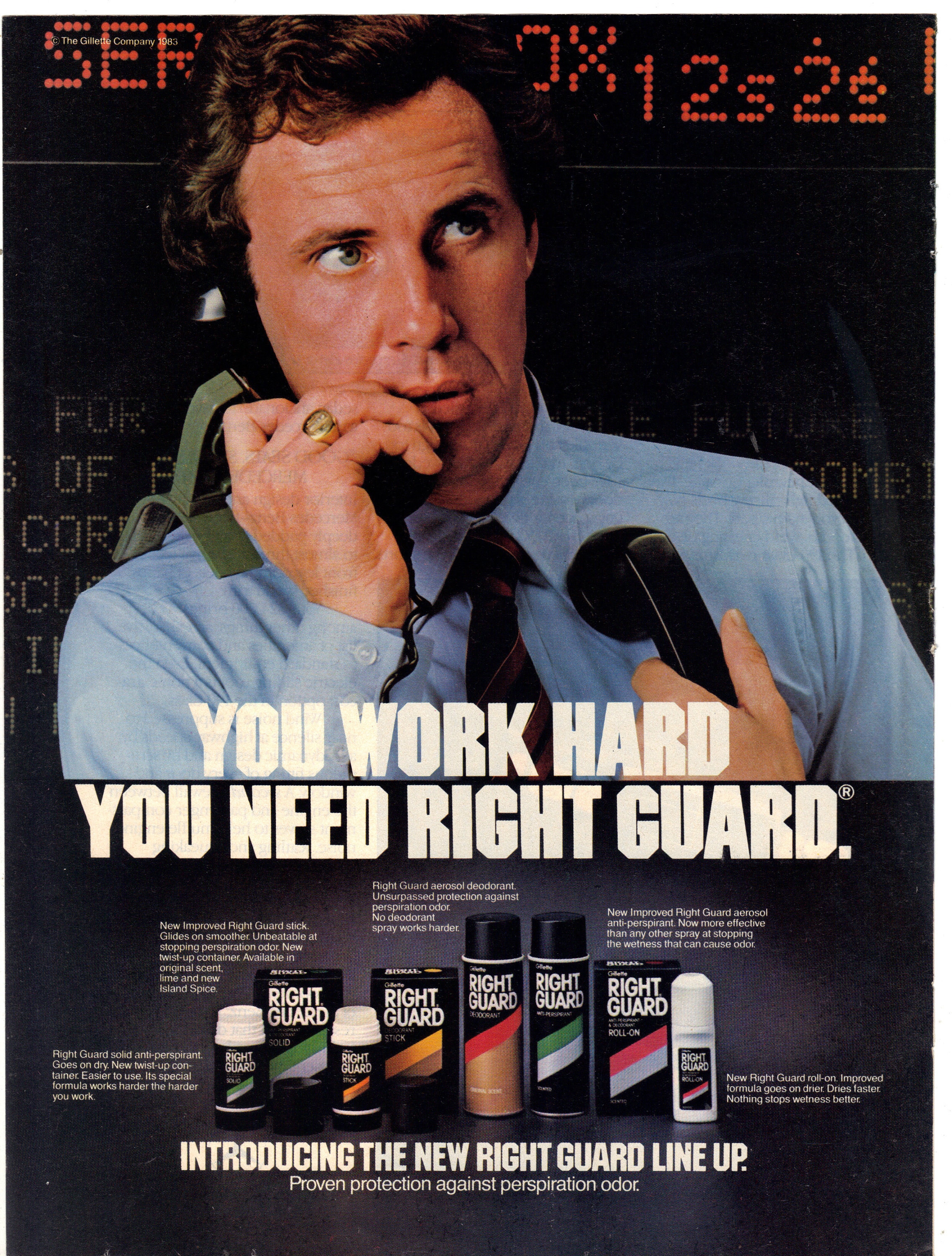The magazine advertisement for RightGuard, likely from the 1980s, features a stockbroker standing attentively in front of a neon stock exchange board. The man, dressed in a blue button-down shirt and a dark tie, sports a short haircut and a gold signet ring on his right hand. He holds an old-fashioned phone receiver to his right ear with the help of a green plastic stand, while his left hand grasps another phone receiver against his chest. The prominent white text at the top reads, "You work hard, you need RightGuard." The bottom of the ad showcases an array of RightGuard products, including aerosol sprays, roll-ons, aftershave, and shaving cream. It concludes with the text, "Introducing the new RightGuard lineup, proven protection against perspiration and odor."